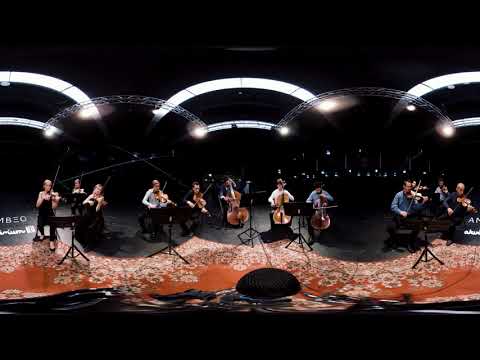In the image, a dozen musicians are performing on a dark-colored stage during a classical music concert. The backdrop and ceiling are black, adorned with designer half-moon-shaped lights that curve slightly at each end, creating a dynamic illumination across the stage. Overhead, silver rafters hold dome-shaped lights casting a white glow. 

The musicians, a mix of male and female artists, are all seated and spread across the stage. On the far left, three women dressed in black play violins. Beside them, two men, one in a blue shirt and another in a black shirt, also play violins. To their right, a person playing the cello is flanked by two additional cellists, all seated and focused on their instruments. The rightmost section features four violinists, two in the front and two behind, adjusting a mix of blue, white, and black attire. 

Each musician has a black music stand in front of them, holding their sheet music. The stage floor is black, while a distinctive red carpet with white floral designs adorns the front section of the stage. The image also features partially visible text reading "M-B-E-O," though it's incomplete. Despite the lack of a visible audience, the detailed setting and the musicians' focused dedication convey the essence of a live classical concert.